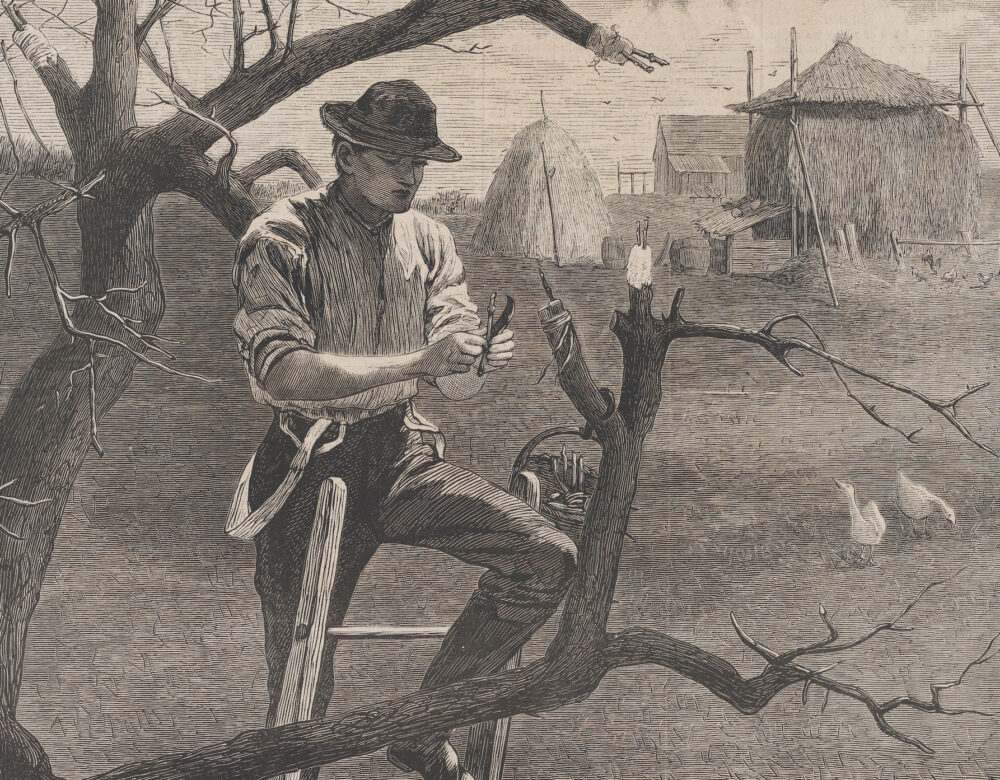This vintage sepia-toned illustration depicts a scene from the late 1800s, showcasing a young farmer perched high on a handmade wooden ladder as he works on a barren tree. Dressed in brown trousers, half-length boots, and a wide-brimmed brown hat, the man wears a white button-up shirt with white suspenders hanging off his shoulders. He appears to be using a rope or string, and possibly a knife, to whittle or cut parts of the tree, with a bucket of implements hanging from a branch nearby.

In the background, there’s a depiction of a rustic farm setting. A large hay bale stands prominently, adjacent to a thatched-roof shack made of straw, which also serves as roosting quarters where chickens are seen pecking at the ground. Further behind, there's a farmhouse. To the right of the tree, two small birds, likely ducks, are visible, adding life to the serene farm scene.